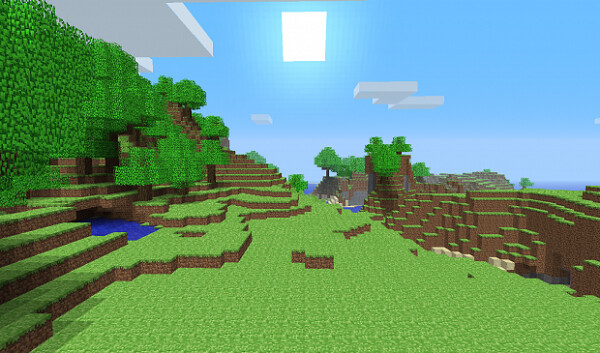The image depicts a vivid game scene set against a bright blue sky, with a distinct pixel-art style. In the center of the sky, there is a bright white square that likely represents the sun, alongside several white flat boxes symbolizing clouds. The background features square, stylized trees, enhancing the game's retro aesthetic. The foreground is dominated by a vibrant green ground cover. Centrally, there are two brown steps overlayed with the same bright green material. On the left, multiple steps ascend a hill surrounded by lush greenery, leading up to a structure with a flat, white roof, partially visible with two distinct sections. To the left of the hill is a gorge, contrasting with the right side where more green covering meets brown land, descending gradually into the distant sky.